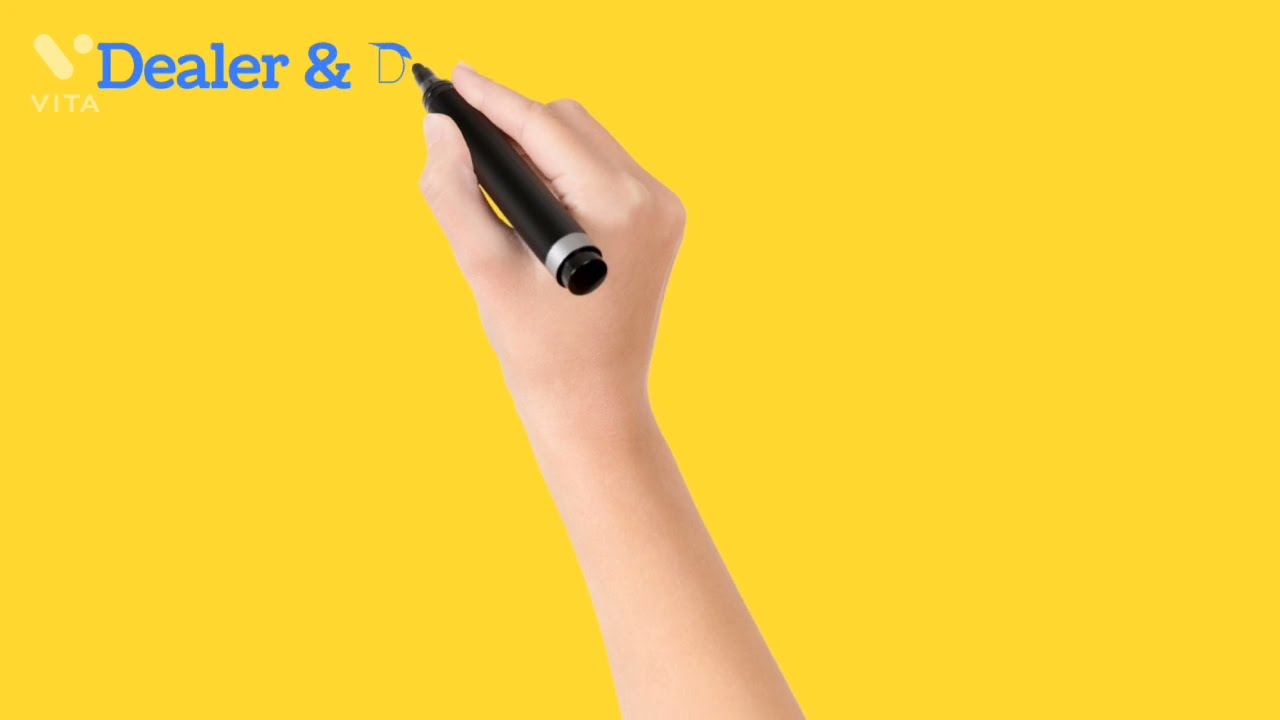The image features a close-up of a hand belonging to a white person, currently writing the letter "D" with a black marker that has a gray strip near its top. The hand, appearing small and possibly that of a child's, is not very hairy, and the fingernails blend in color-wise with the skin. The background is a flat, darkish yellow, entirely unadorned. In the upper left corner, there's white text spelling "VITA" in all capital letters, beneath a small white logo resembling a sideways cylinder with a dot to its right, forming the stylized shape of a "V." Adjacent to "VITA" is the word "dealer" in blue lowercase letters, followed by an ampersand, and then the hand is seen writing the second "D" in a word that is yet to be fully revealed. This composition gives the impression of an advertisement, possibly for a product or brand name, likely a screenshot from a commercial or a webpage.